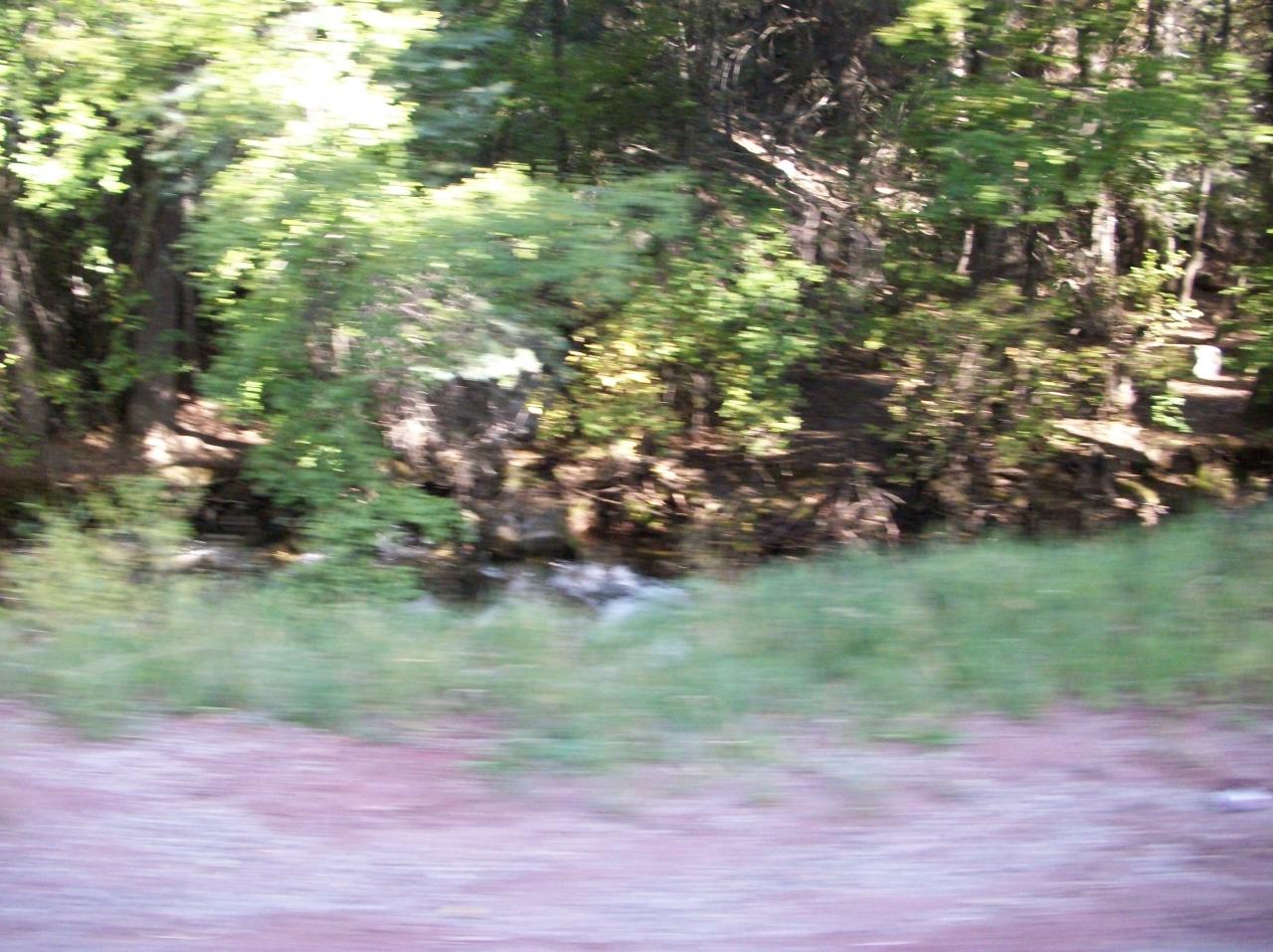In this somewhat blurred image, the bottom portion features a light pinkish or purplish-brown tint, resembling dirt or soil, interspersed with lighter patches that could be rocks. Above this, a layer of green textured plant life spans from left to right, suggesting grass or low-lying bushes. Further up, there is what appears to be a dense forest area with tall green trees, with more branches, twigs, and leaves, particularly noticeable on the right side. A light source illuminates a portion of the left side, creating a mix of shadows and highlights, enhancing the sense of depth in the scene. The entire image has a somewhat indistinct, almost painterly quality, making it difficult to discern specific details.